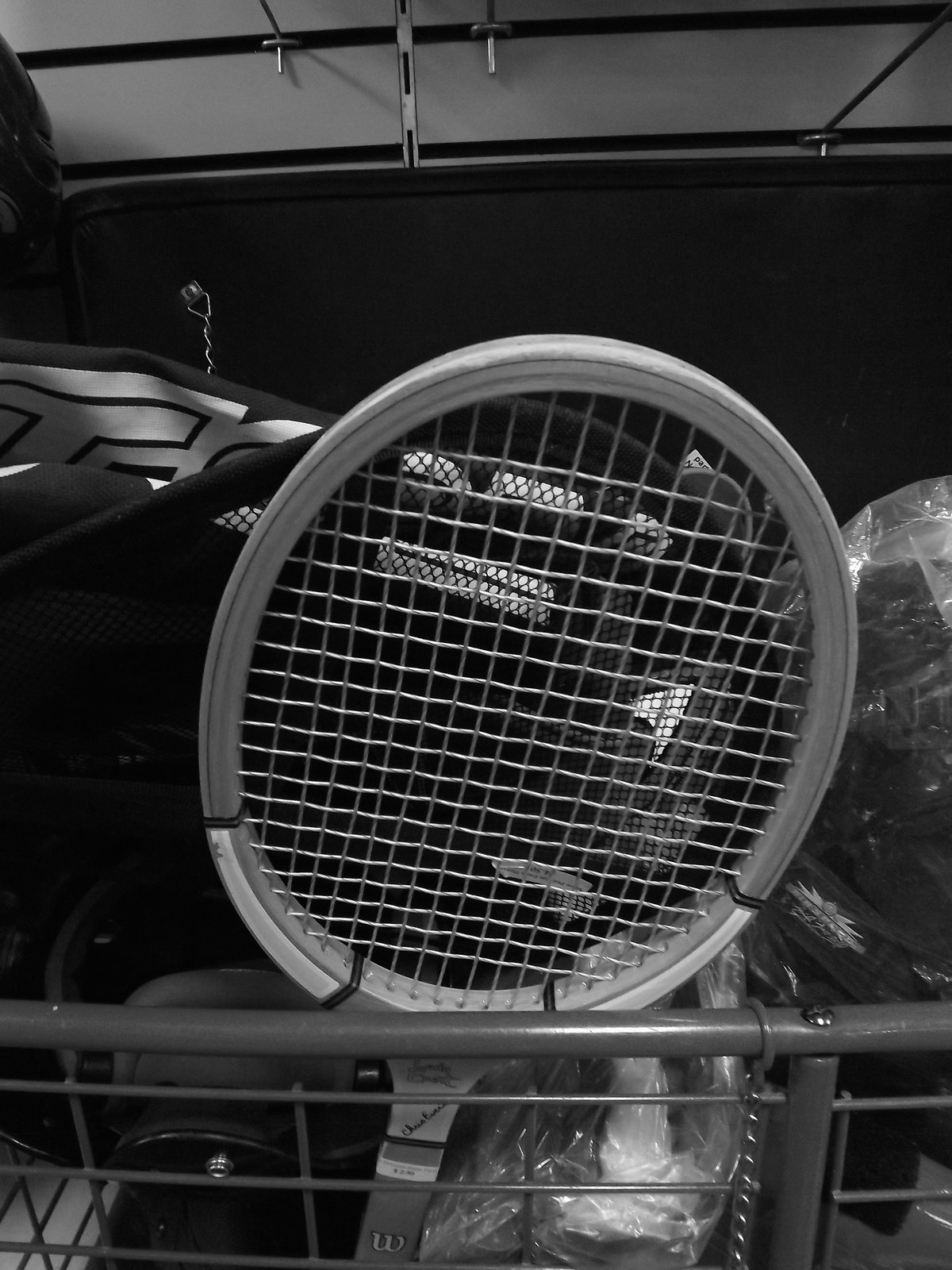This black and white photograph features a detailed scene centered around a tennis racket. The racket, which is gray and dark gray with a distinguishable "W" and an unreadable signature on it, is securely positioned inside what appears to be a metal holder or wire basket. Beneath the racket, there is a plastic bag, possibly containing knee pads, and another object that is partly obscured but identified by a letter "T" in white and black. The background includes black canvas with gray design patterns, suggesting a storage unit setting. Also visible are metal chains hanging off to the side. Above the setup, the ceiling with its distinctive white color and black lines can be seen.